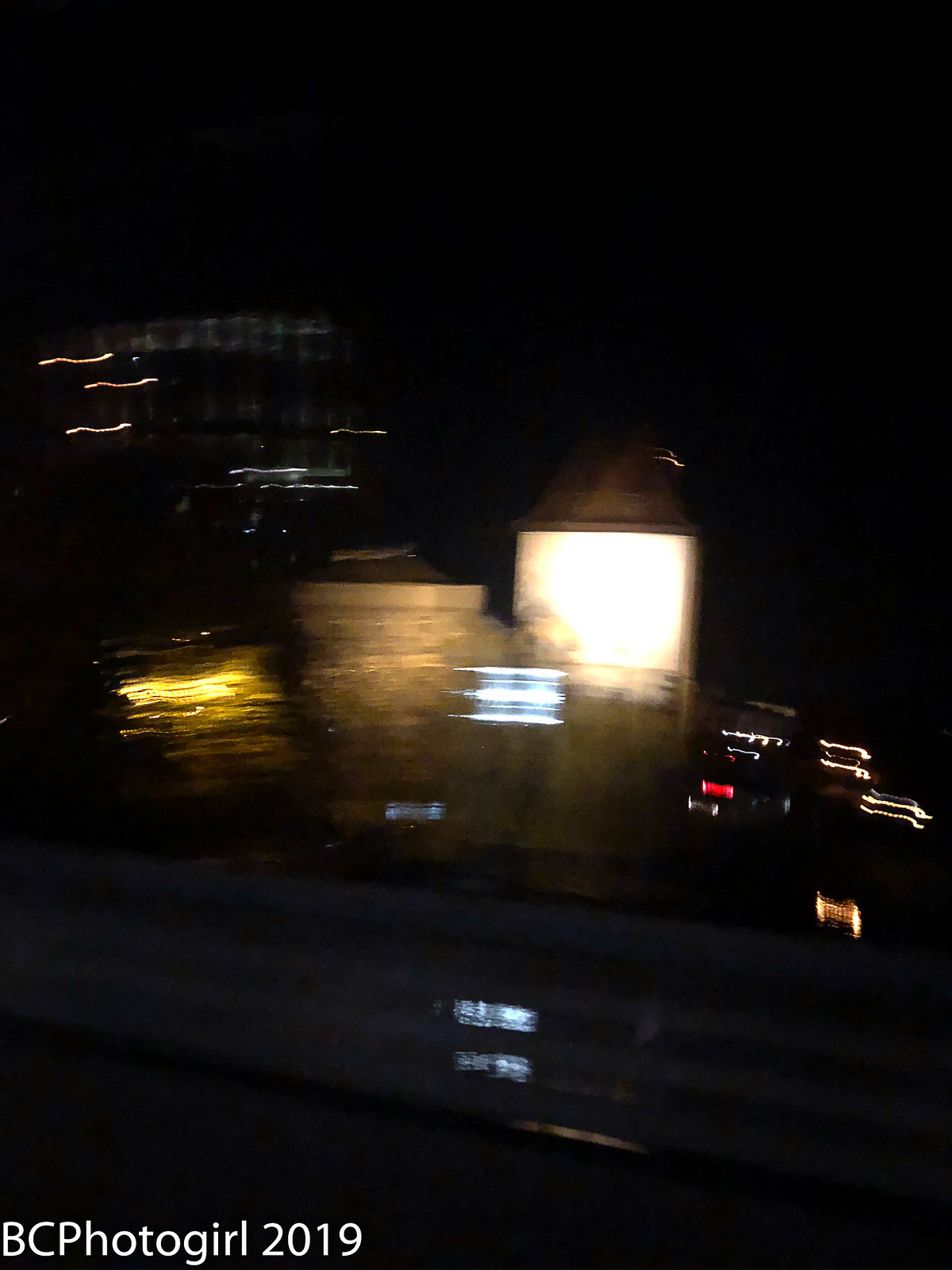A photograph taken at night depicts a scene with several indistinct elements due to the image being blurry. The sky is completely black, indicating nighttime. In the bottom left-hand corner, there is a white watermark that reads "BCPHOTOGIRL 2018." At the center of the image stands a white house or building with a prominent white light. To the right, three buildings of varying heights are visible, the tallest of which is well-lit at the top with a white light, while the leftmost building is dimly lit by a warm yellow light. Scattered throughout the scene are various lights: red and white lights likely from cars, and yellow and white lights that seem to emerge from statues or other objects. To the right of the main structures, there's an array of colored lights (red, orange, yellow, and blue) suggesting the presence of boats. In front of the buildings is a platform with a white wooden fence or ledge. Further back, another building with dim blue lights can be discerned.